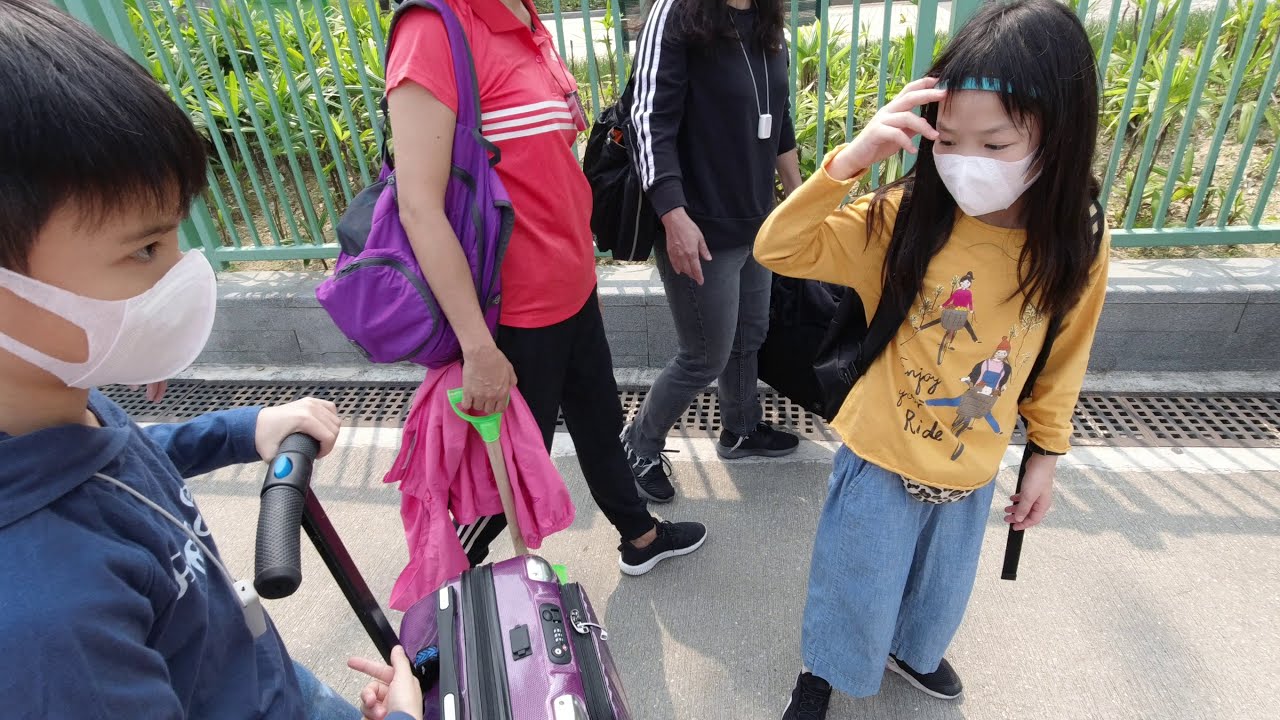The image captures four people traveling together on a sidewalk. In the forefront, on the left side, is a young boy around eight years old, dressed in a blue hoodie and blue jeans. He is pushing a rolling suitcase with purple sides and a combination lock on top. The boy also wears a white mask on his face and grips the suitcase handle with one hand while pointing at it with the other. To his right, a young girl, also wearing a white mask, is dressed in a gold-yellow t-shirt featuring a graphic of two people riding bicycles, blue jeans, and black shoes. She has a black backpack on her back and appears to be looking down at the boy's suitcase or handle.

In the background are two adults walking, partially visible from the shoulders down. The adult on the left wears a red polo shirt with white stripes, black pants, and black tennis shoes while carrying a purple backpack. The person next to them is dressed entirely in black, including a black sweatshirt, black jeans, and black shoes, and also has a black backpack. Both adults are walking in the same direction as the children, creating a cohesive sense of movement and travel.